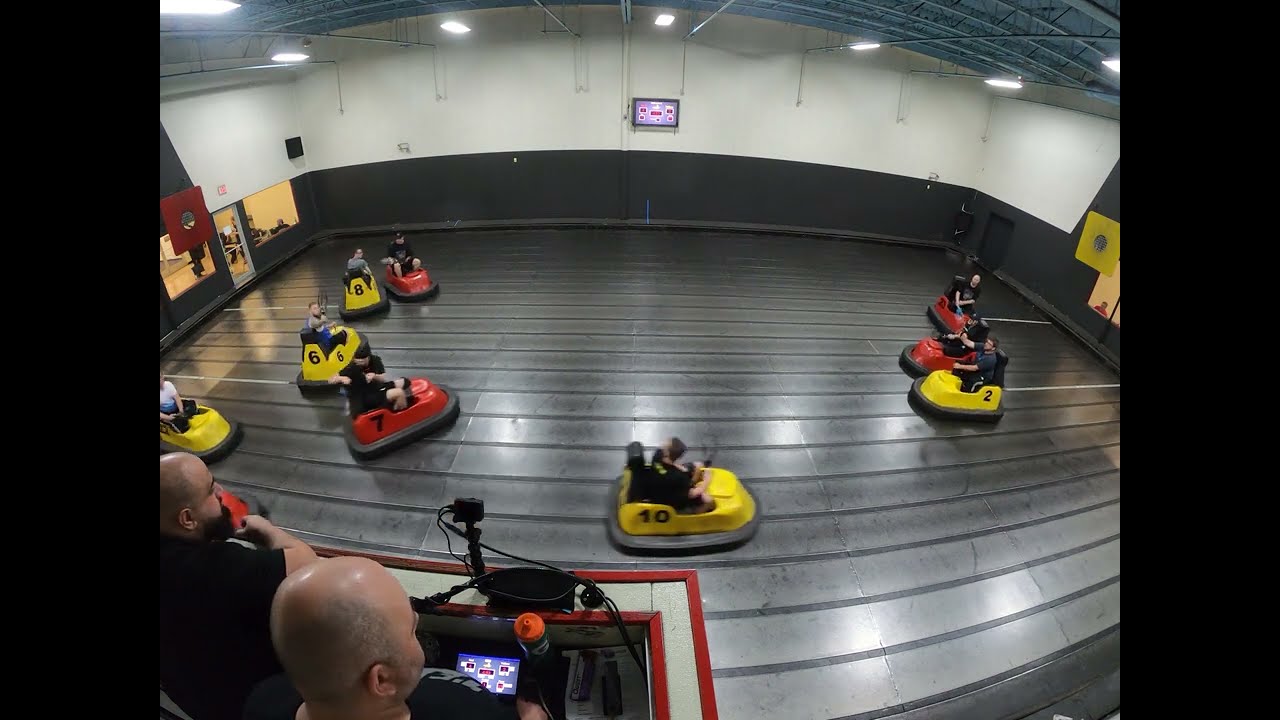The image shows a vibrant indoor bumper car arena with a total of nine cars—five yellow and four red—all driven by adults. Each car is clearly marked with a number: the top left car is numbered 8, the one below it is numbered 6, the center bottom one is numbered 10, and the car on the right displays a 2. The bottom left car’s number is obscured from view. The arena is illuminated by fluorescent ceiling lights, creating a well-lit environment for the activity. 

At the lower left corner of the image, two bald men, presumably judges or supervisors, stand on a platform. One is focusing on a small screen, possibly for monitoring the event, and there's a digital camera positioned to oversee the bumper car floor. The rectangular arena includes structural supports with an arch in the rear and has white walls accented with doors and windows near the goal lines on both sides. A scoreboard is mounted at the center but is not clearly readable. Beyond the immediate bumper car area, a bench with onlookers or participants waiting can also be seen. This electrifying sport, powered by battery-operated bumper cars, takes place on a glossy black floor that might suggest a hovercraft-like mechanism.